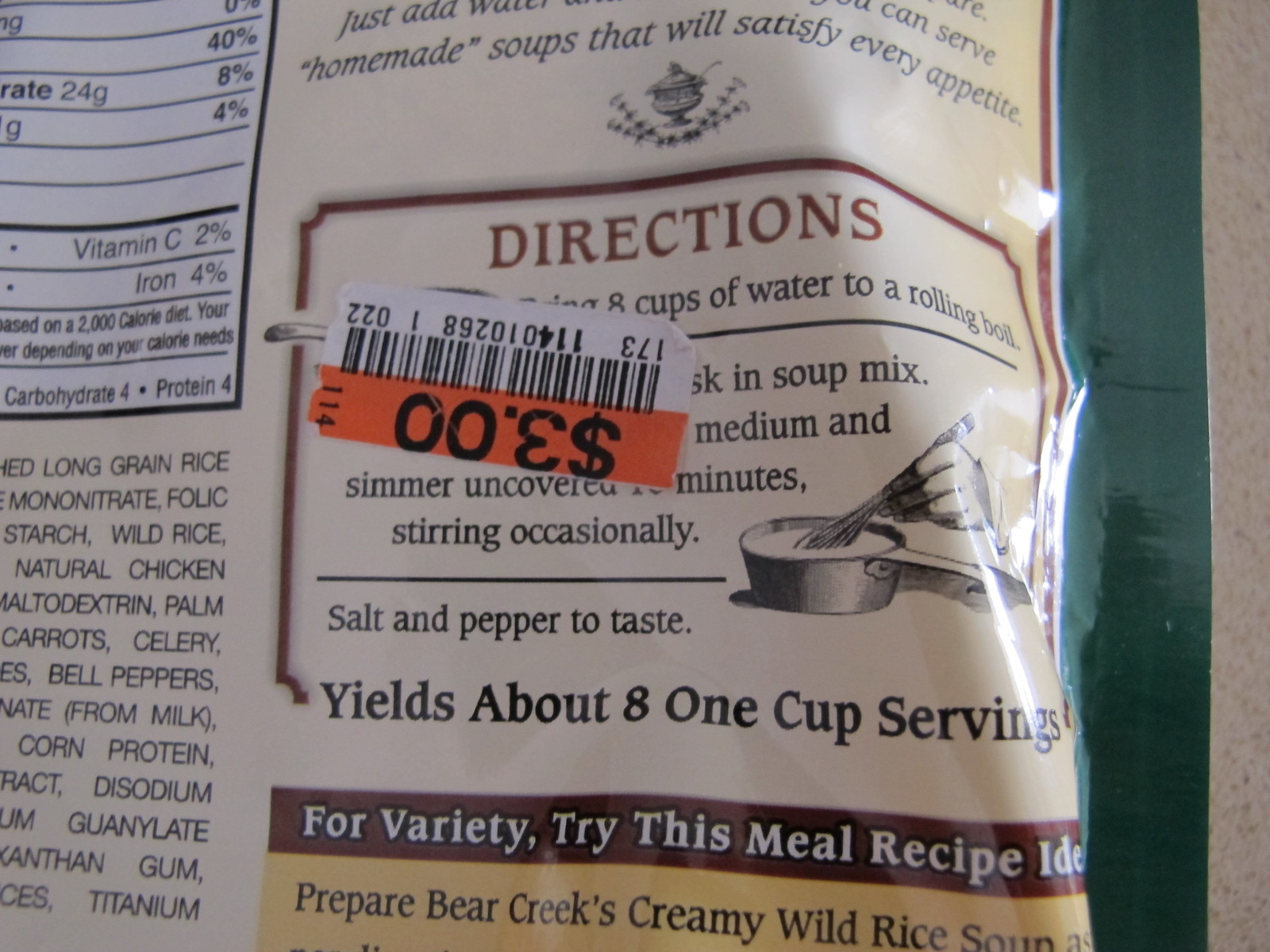This is the back of a Bear Creek's Creamy Wild Rice Soup package. The photo shows the instructions for preparing the soup, though they are partially obstructed by an orange clearance sticker with a $3 price tag and a barcode. The visible instructions suggest bringing eight cups of water to a rolling boil, whisking in the soup mix, simmering on medium heat, stirring occasionally, and seasoning with salt and pepper to taste. This yields about eight one-cup servings. To the upper left, the nutrition information is partially visible, displaying percentages such as 40%, 8%, 4%, and 2% for Vitamin C. The lower left-hand corner contains a partial list of ingredients, including long grain rice, wild rice, maltodextrin, palm protein, chicken stock, celery, carrots, bell peppers, and corn protein. The package also offers a meal recipe idea for variety. The background reveals the package resting on a countertop.